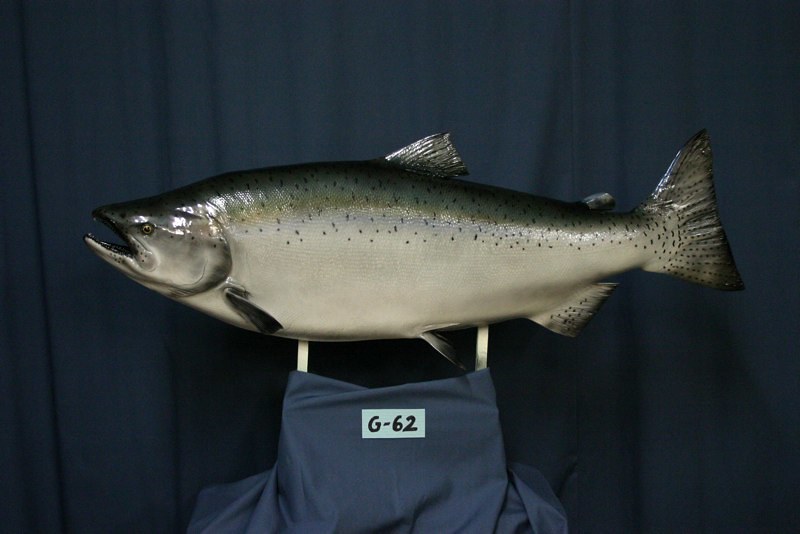This photograph features a large, meticulously detailed fish, which appears to be either a sculpture or a taxidermy specimen mounted on two metal bars. These bars are wrapped in a blue cloth matching the dark blue, curtained backdrop. Taking up most of the frame, the fish is centered prominently, pointing to the left with its mouth open and eyes frozen, gazing downward. It has a small dorsal fin on top, a proportional fan-shaped tail, and an additional lower fin near its tail. The fish exhibits a gradient coloration: its silver body darkens at the top, speckled with scales, transitions into a lighter gray towards the middle, and ends with a white underbelly. Various shades of brown, gray, and black add nuances to its upper part, complemented by white lighting reflecting off its scales. The setup also includes a label marked "G62" attached to the blue material around the metal frame.